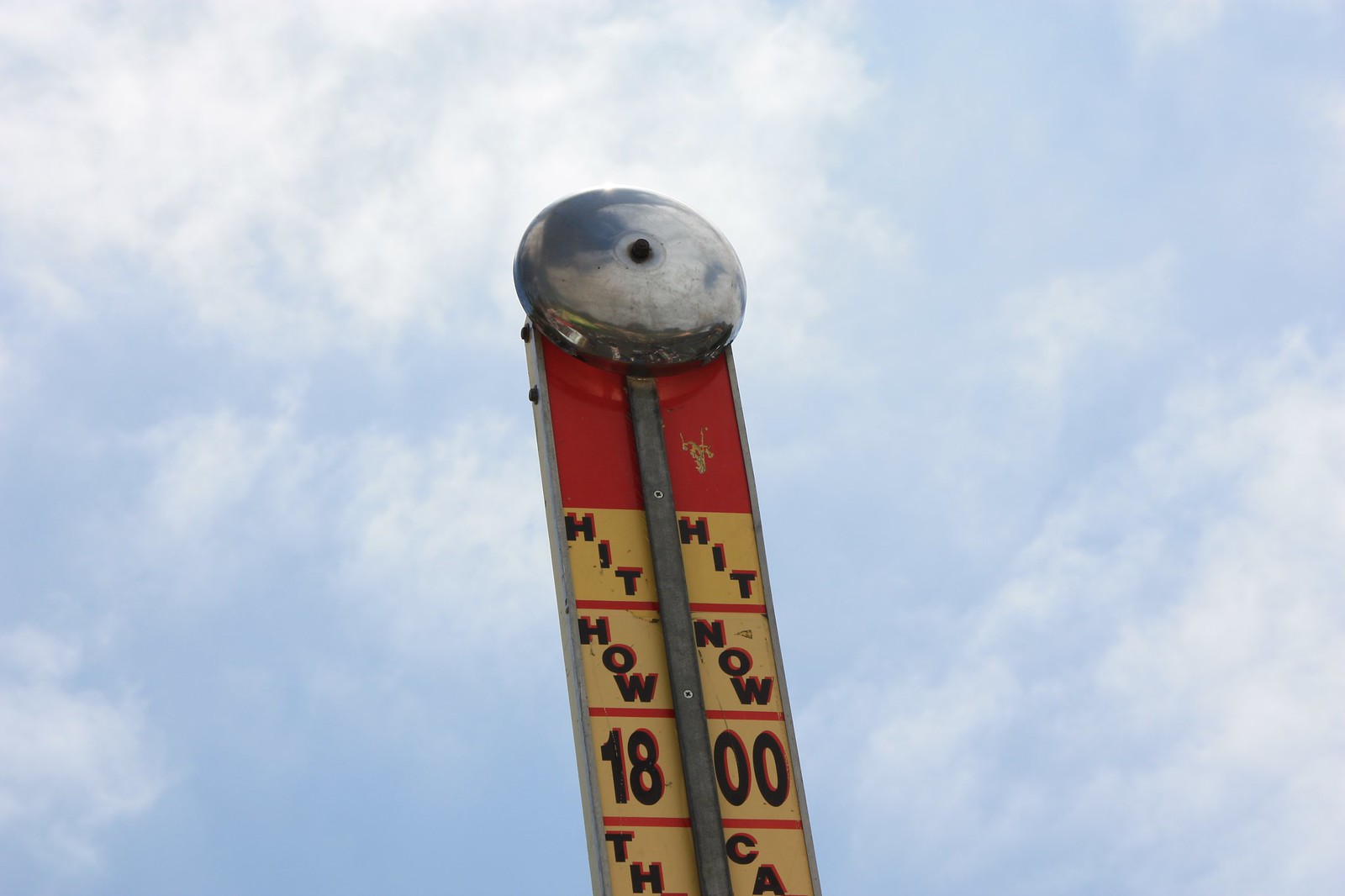The photograph captures a classic carnival game, specifically the strength test where participants use a large rubber mallet to hit a pad, propelling a weight up a vertical track in an attempt to ring a bell. The top portion of the game board is visible, showcasing the vintage bell and the weathered track that the weight climbs. Below the bell are various markings, including "1800," "HOW NOW," "HIT HIT," and other partially visible letters, indicating the different levels of achievement for players.
 
The vintage nature of the game is evident in the worn wood of the vertical backboard and the rusted bolts holding the bell in place, suggesting the game has been a mainstay at many carnivals over the years. The backdrop features a fair-weather sky with light blue hues and puffy clouds, adding to the nostalgic ambiance of the scene. The entire setup, from the aged materials to the design, evokes a sense of timeless fun and challenge at the fairground.